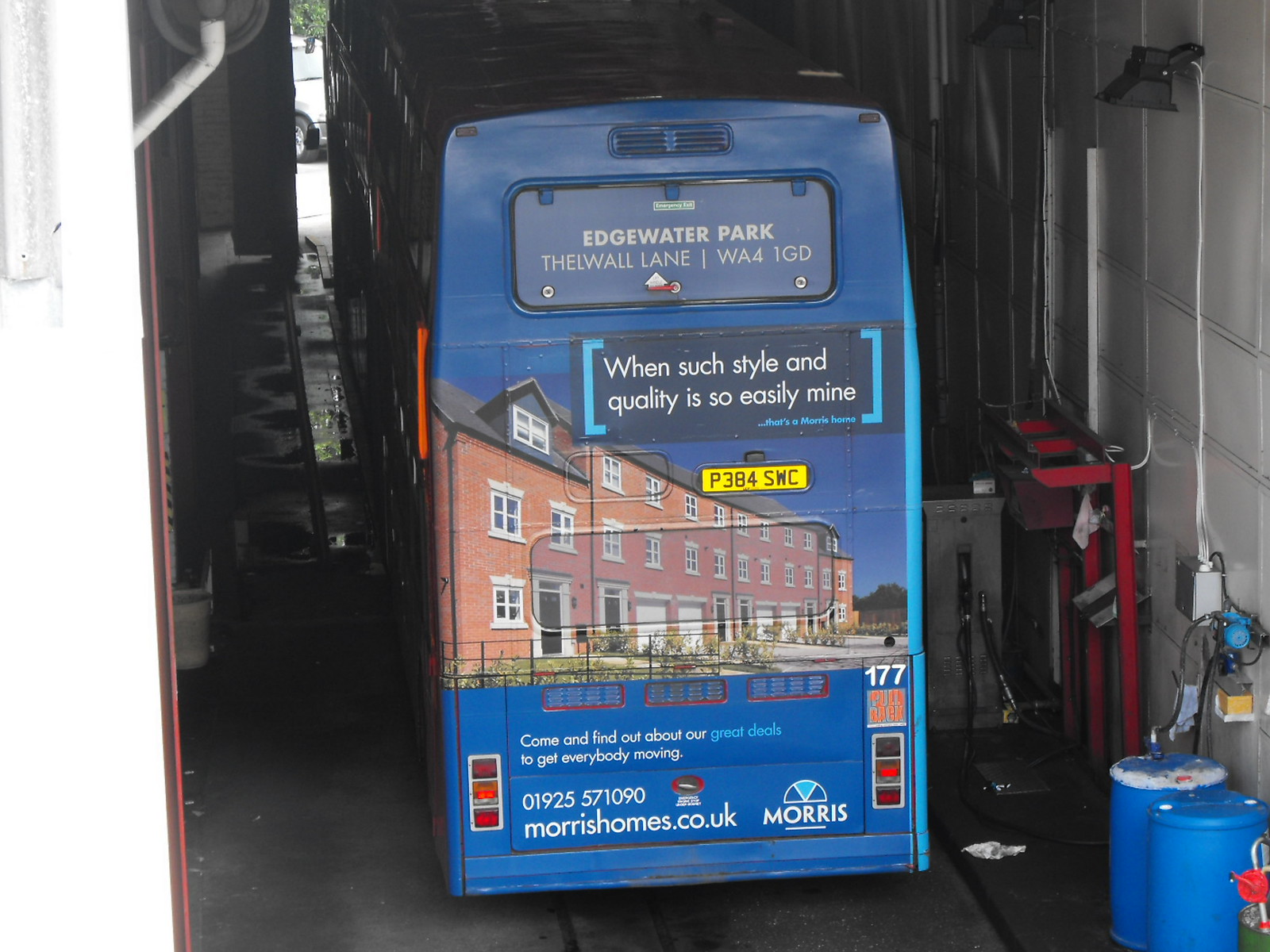In a dimly lit garage where vehicles come in for repair or maintenance, a towering blue double-decker bus stands out against the surroundings. 

The bus is positioned on a track, perhaps for a bus wash, with puddles of water visible on the ground. The back of the bus is prominently displayed, featuring a comprehensive advertisement that covers the rear windows. The advertisement showcases a large, elegant black-brick manor with white windows and a black roof, possibly an old-style hotel or apartment building. Above the image of this building, the text reads, "Edgewater Park, Thelwall Lane, WA41GD." 

Midway up the bus, just below the advertisement, there’s a license plate marked "P384SWC." Prominently, the ad bears the tagline, "When such style and quality is so easily mined," encouraging viewers to "come and find out about our great deals to get everyone moving." At the bottom of the advertisement, the text directs interested parties to MorrisHomes.co.uk, featuring the Morris Homes logo.